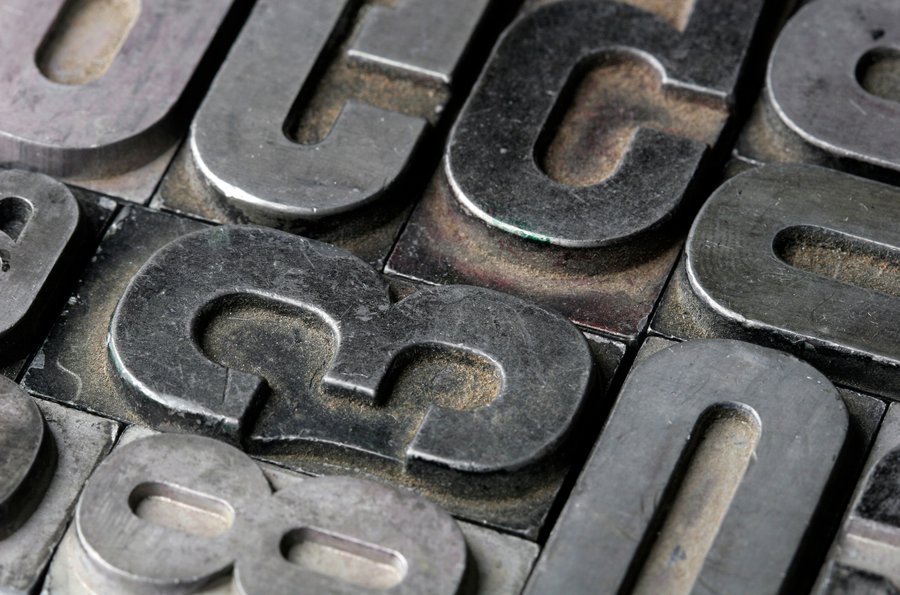The image is a close-up, partially cropped, and zoomed-in view of several metal pieces, appearing to be a collection of letters and numbers. The characters are raised and seem to be large, with distinct variations in their shades of metal—some light, some dark. This diversity in shades highlights their worn-out, possibly rusted, and dirty condition. Key identifiable characters include the numbers 3, 5, 8, and 0, as well as letters such as U and C. The metal pieces are randomly arranged, pushed side by side, with no clear order. The purpose of these characters is somewhat ambiguous, but they might be used for printing, where ink is applied over their raised surfaces, or potentially for branding on materials like leather, given their metallic nature and prominent raised design.